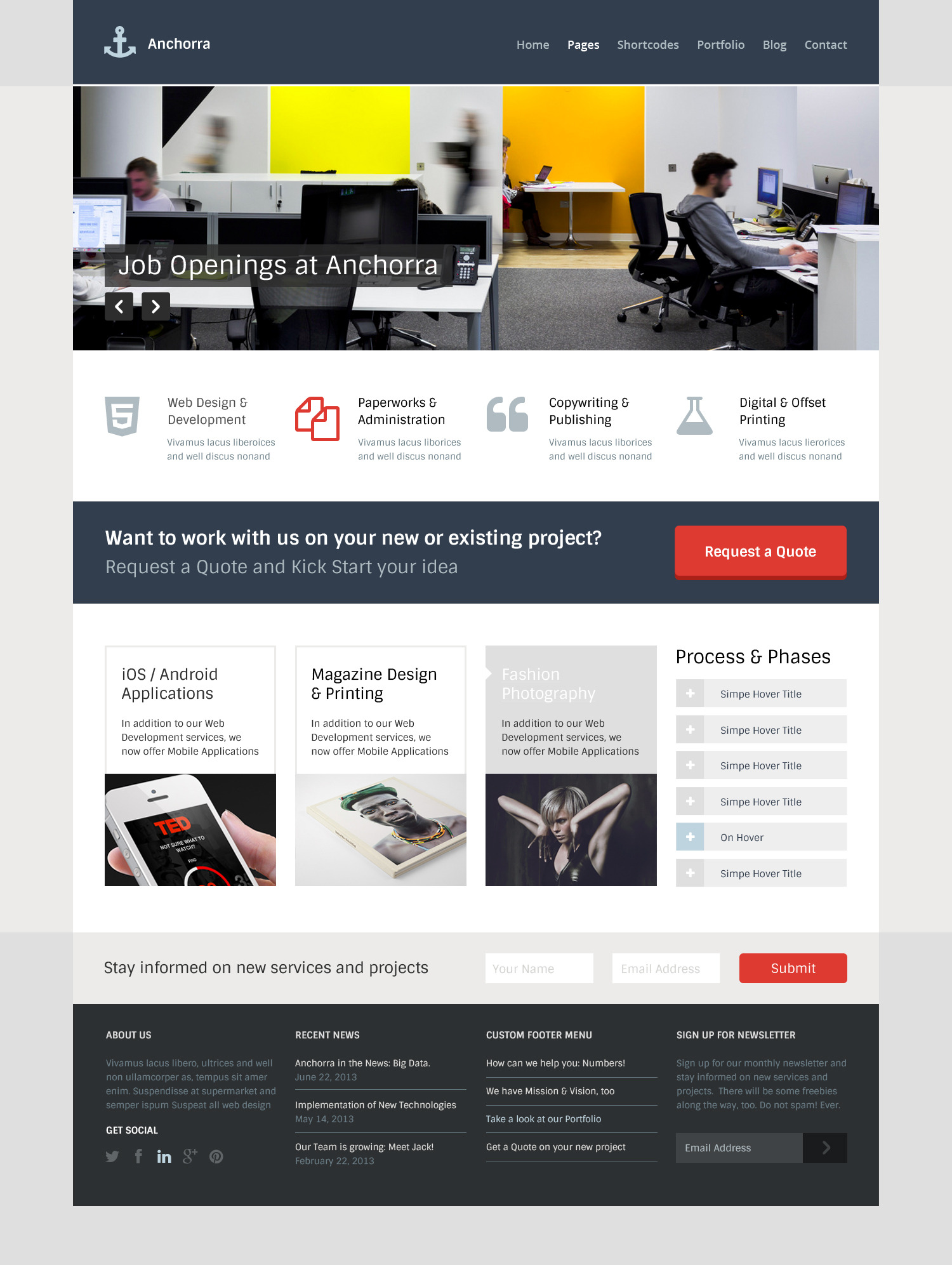The image depicts a blurry, low-resolution webpage with a dark blue background. At the top left, there is a light blue artwork of an anchor, adjacent to the word "Anchora," spelled "A-N-C-H-O-R-A" in white text. To the right of the logo, there are six navigation tabs labeled: Home, Pages, Shortcodes, Portfolio, Blog, and Contact. Below the navigation, the text "Job Opening at Anchora" is visible. The background features an office scene with several people. On the right side of the image, a man is sitting on a black chair at a desk, working on a monitor. Beneath the main text, there are additional labels from left to right, specifying job roles: Web Design and Development, Paperwork, and Administration.